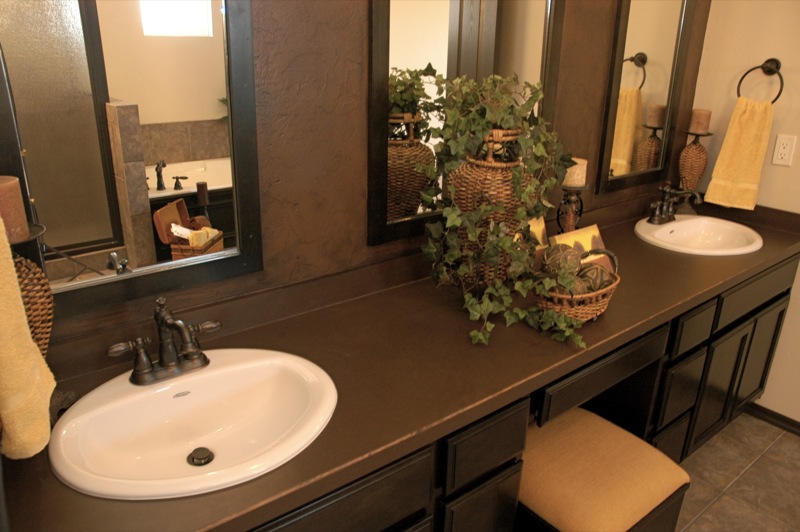This image showcases an opulent bathroom characteristic of an upper-class establishment. Prominently featured are two antiquated sink faucets, each a distinct brownish-black color, mounted on pristine white sinks positioned on either side of the frame. The photograph, taken at an angled perspective, reveals the slightly smaller right sink on the right side and the left sink near the bottom left corner of the image. Flanking each sink are towels in a tannish-yellow hue, enhancing the vintage ambiance.

An electrical outlet is visible on the wall beside the right sink. Centered on a brown table that supports the sinks sits a decorative vase, possibly crafted from leather-like material, brimming with verdant green leaves. This table, adorned with numerous square and rectangular drawers, offers ample storage. Below the table and between the sinks, a backless chair with a tannish cushion is nestled, adding to the room's functionality and elegance. Behind the sinks, mirrors affixed to the wall capture reflections of the lavish environment, adding depth and a touch of grandeur to the overall aesthetic.